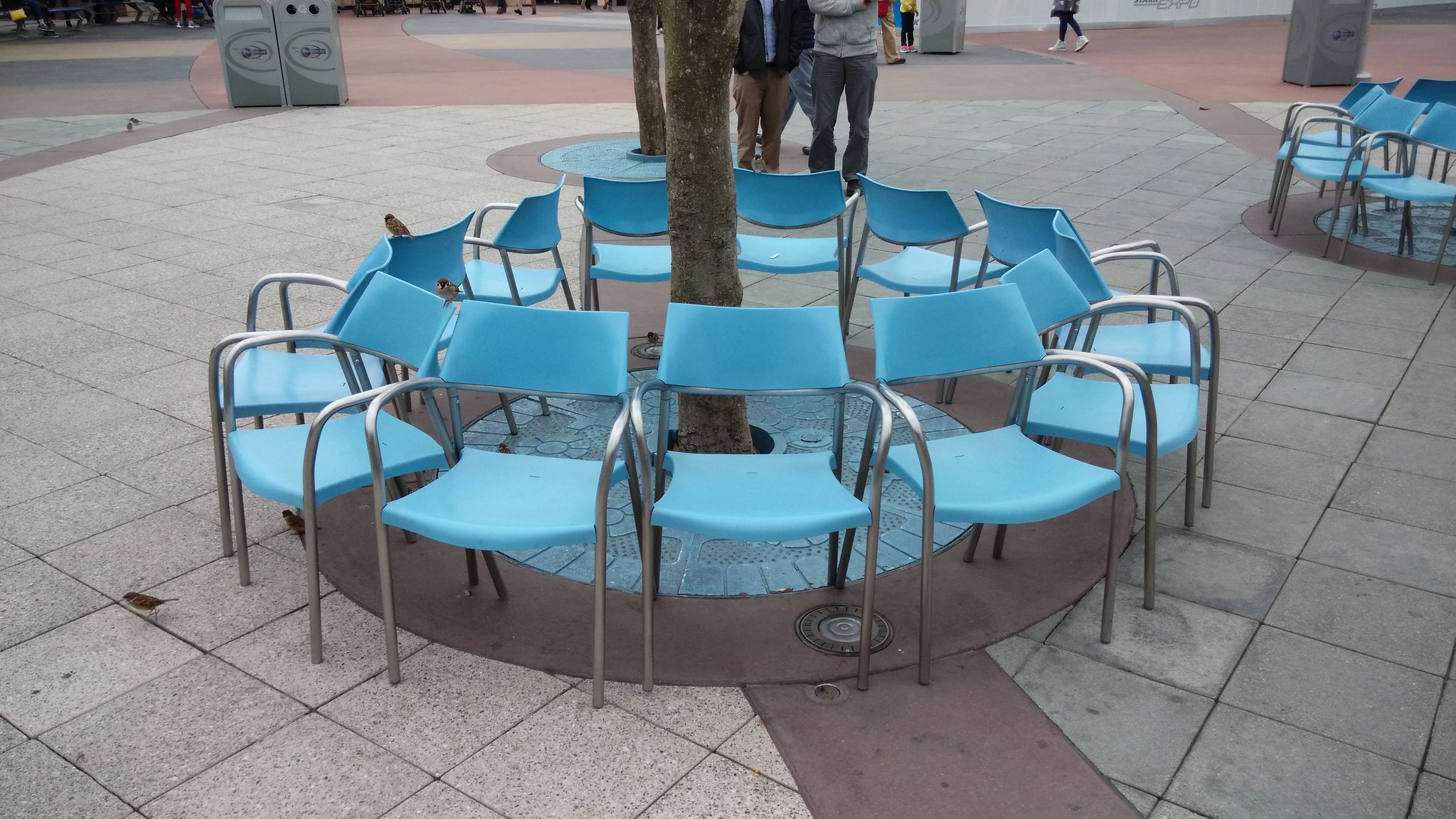The photograph captures a lively seating area in an urban or park setting, showcasing a meticulously designed stone-paved floor. The paving consists of square-shaped concrete tiles in shades of white, slightly pink, and grey, with accentuating dusky red stonework encircling certain features. Central to the image is a tree, its trunk surrounded by a grate and a decorative circular arrangement of pink concrete detailing.

Encircling the tree are 13 blue chairs, their seats and backs seemingly made of canvas, with silvery tubular metal arms that seamlessly become the legs. Each chair faces outward from the tree, creating a communal but spaced-out arrangement. To the right of this central tree, another similar arrangement of blue chairs hints at yet another tree, unseen in this portion of the photograph.

The background features indistinct figures wearing muted tones of brown, grey, and black, captured from the chest down, with one person notably crossing a road visible at the top of the image. Additionally, small birds perch on the backs of two chairs and are scattered around the ground near the tree, adding a touch of life to the scene. Machinery and garbage cans for recycling and regular trash can also be spotted in the farther reaches of the photo, contributing to the everyday urban backdrop.